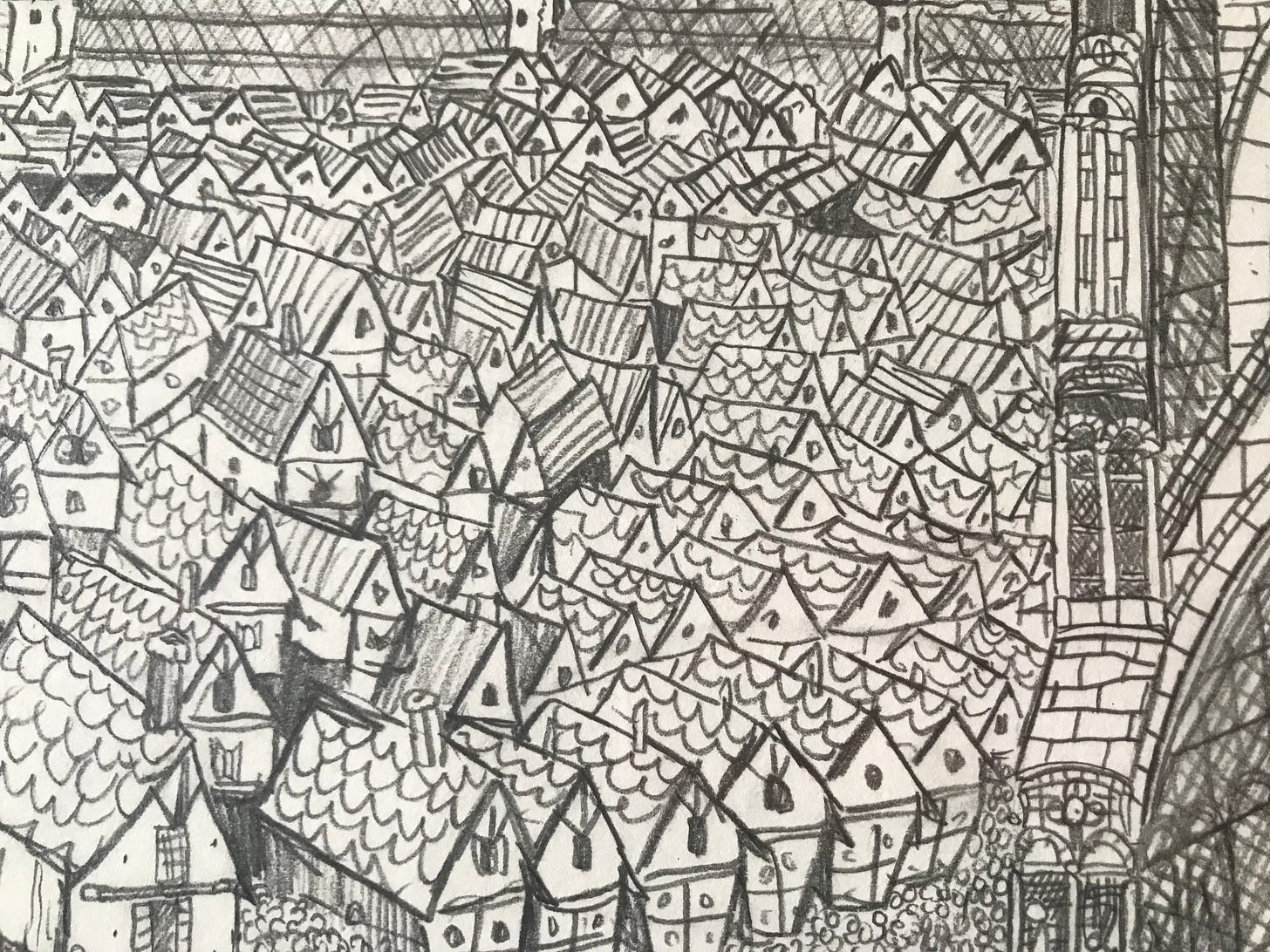This detailed square pencil sketch portrays a bustling aerial view of a dense collection of houses, likely set in a medieval European town. The rooftops, identical in their three-dimensional triangular shapes, dominate the image with squiggly and shaded lines indicating the roof shingles. Circles depict windows on the facades. The variety in the rooftops, some featuring chimneys while others do not, adds to the complexity of the scene. On the right side, a larger structure, possibly a church, stands out with its distinctive windows. In the top background, zigzagging lines with posts suggest the presence of fencing, while a possible train is hinted at descending from the top right. The entire drawing is meticulously filled with intricate details, showcasing even the smallest pencil strokes, capturing a beautiful and very busy medieval townscape.